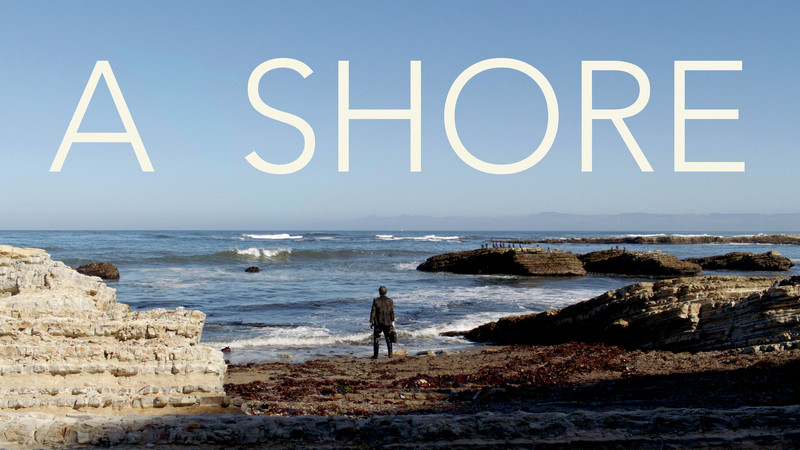In this detailed photo, we see a captivating coastal scene primarily focused on a shoreline. The image, rectangular in shape, features a man standing with his back to the camera towards the bottom center. He is positioned on the edge of a rocky beach, gazing thoughtfully out at the ocean, with waves gently rolling in around him. The scene includes an array of colors: the serene blue of the water, the white of the waves, and various shades of gray, brown, tan, and light brown from the rocks and shore. At the top of the image, there is text in large, white, cream-colored capital letters that reads "A SHORE." The entire composition has a contemplative atmosphere, suitable for use on a postcard or blog, evoking a sense of calm and introspection typical of someone in deep thought, surrounded by the vast and beautiful coastline. The photo’s angle, taken from behind the subject, emphasizes the expansive seascape and rugged terrain, perhaps even suggesting distant mountains and faint figures further away.